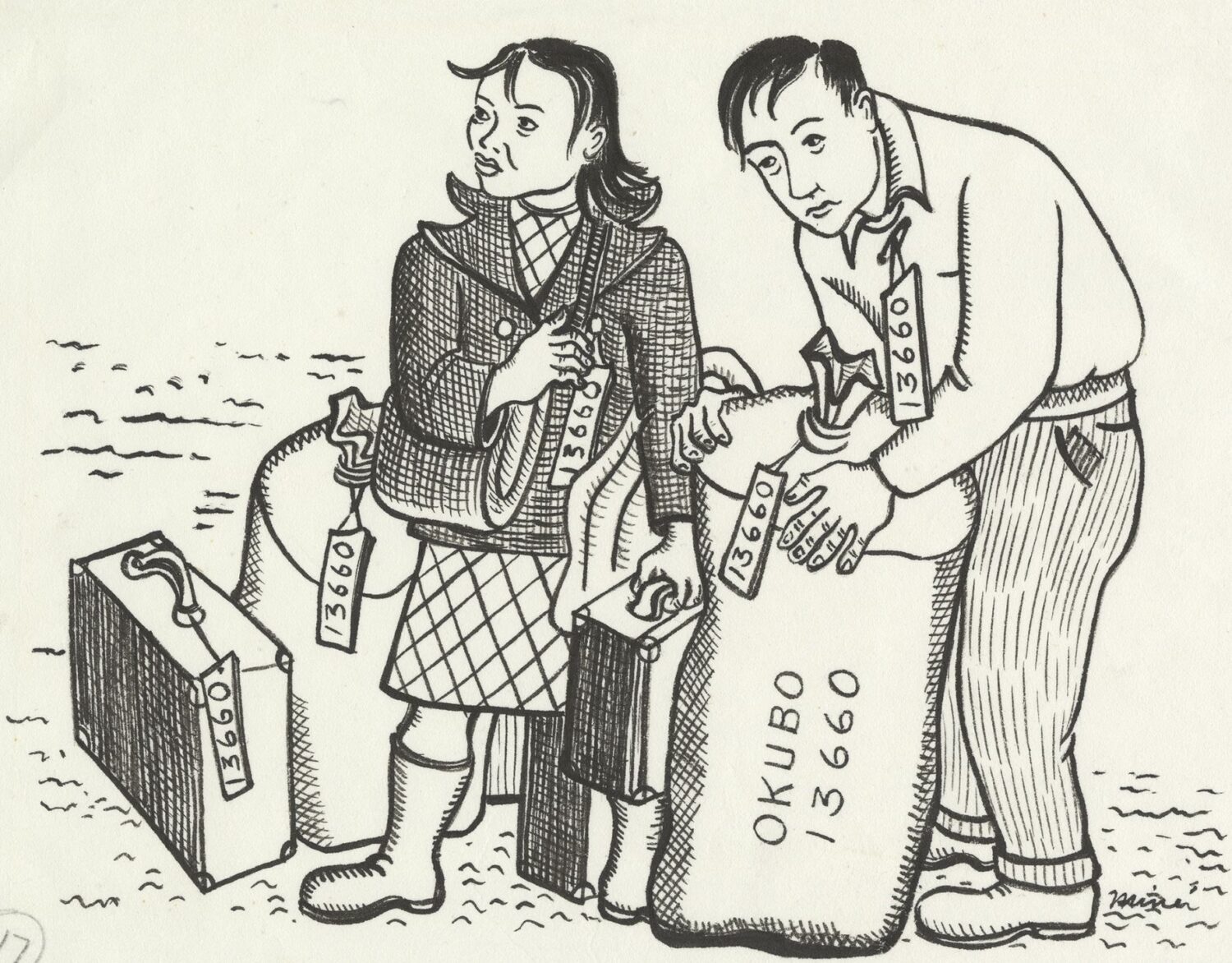This black and white sketch art drawing depicts two likely Asian immigrants with their luggage, potentially arriving from sea. The woman, who is possibly in her 30s or 40s, is wearing a short plaid skirt, knee-high white rubber boots, a button-up jacket, and has a purse slung over her shoulder. She is facing towards the left side of the image and is holding a suitcase in one hand. Surrounding her are several suitcases and bags, all labeled with the number 13660.

Behind her, to her right, is a man wearing a collared, long-sleeve shirt, striped long pants, and white shoes. He is also likely in his 30s or 40s. The man is hunched over, clutching a large sack with both hands that is labeled "OKUBO 13660." Both individuals have tags with the number 13660 attached to their clothing, matching the numbers on their luggage. The scene is set against a light gray background and captures the essence of their immigrant status through meticulous and thoughtful sketching.